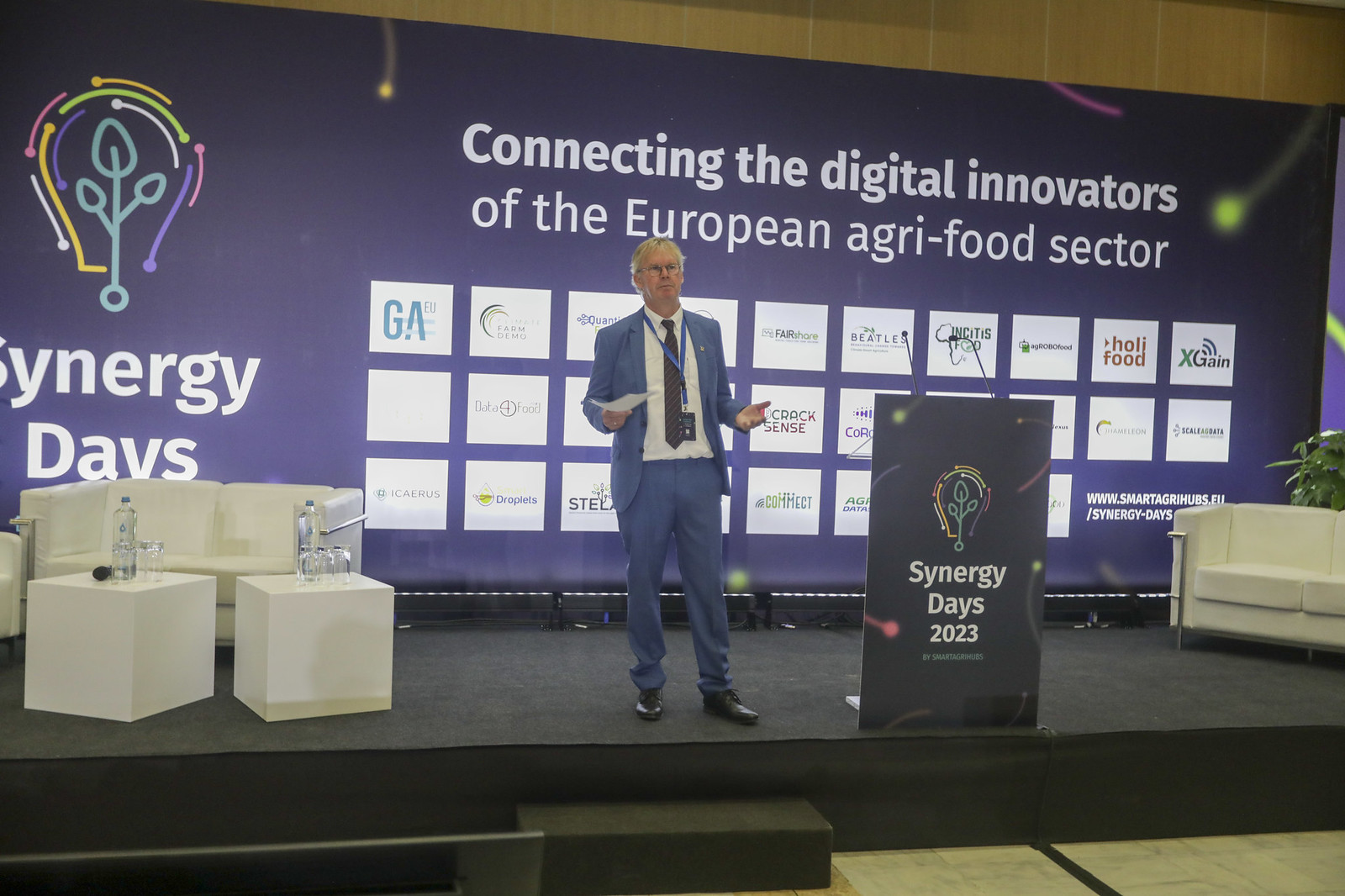In this detailed image, a man is standing on stage delivering a speech at an event called Synergy Days 2023. The stage has a dark tone, and the backdrop is a striking dark blue featuring colorful swirling star designs in pink, yellow, and blue. The backdrop displays a large projected message that reads, "Connecting the Digital Innovators of the European Agri-Food Sector," with rows of sponsor logos below, partly obscured but including names like xGain, Halifood, and GA. The Synergy Days logo, a plant with three branches encased in light bulb-like lines, is prominently featured.

The man is positioned beside a black podium marked with "Synergy Days 2023" in white letters, equipped with microphones. He is dressed in a blue suit, white collared shirt, dark tie, and black shoes, accessorized with glasses and a lanyard, and has short gray hair. His hands are raised, palms up, possibly holding a paper. 

On the left side of the stage, there's a white loveseat with two cube-shaped white tables in front of it, each holding a water bottle. The right side of the stage contains a tan couch and similarly styled furniture.